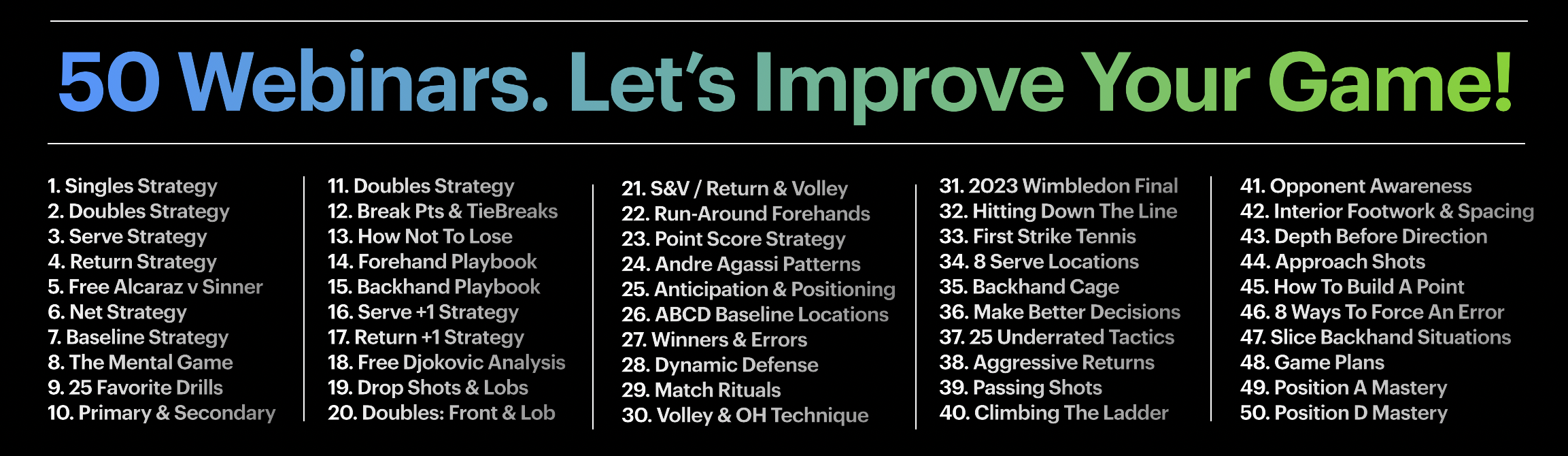The image depicts a detailed list designed to aid in game improvement, titled “50 Webinars: Let's Improve Your Game” in vibrant text that transitions from blue to green. The background is black, and the list is methodically organized into five columns, each separated by thin white vertical lines. The list is numbered in white and is introduced by white horizontal lines above and below the main title. The top ten topics underline crucial aspects such as Single Strategy, Double Strategy, Serve Strategy, Return Strategy, Free Alcarez v. Sinner, Net Strategy, Baseline Strategy, The Mental Game, 25 Favorite Drills, and Primary and Secondary Strategies. This list offers comprehensive strategies and tips, covering various elements of gameplay including opponent awareness, interior footwork and spacing, depth before direction, approach shots, and methods to force errors. The structured presentation and exhaustive content aim to enhance every facet of the player's game.